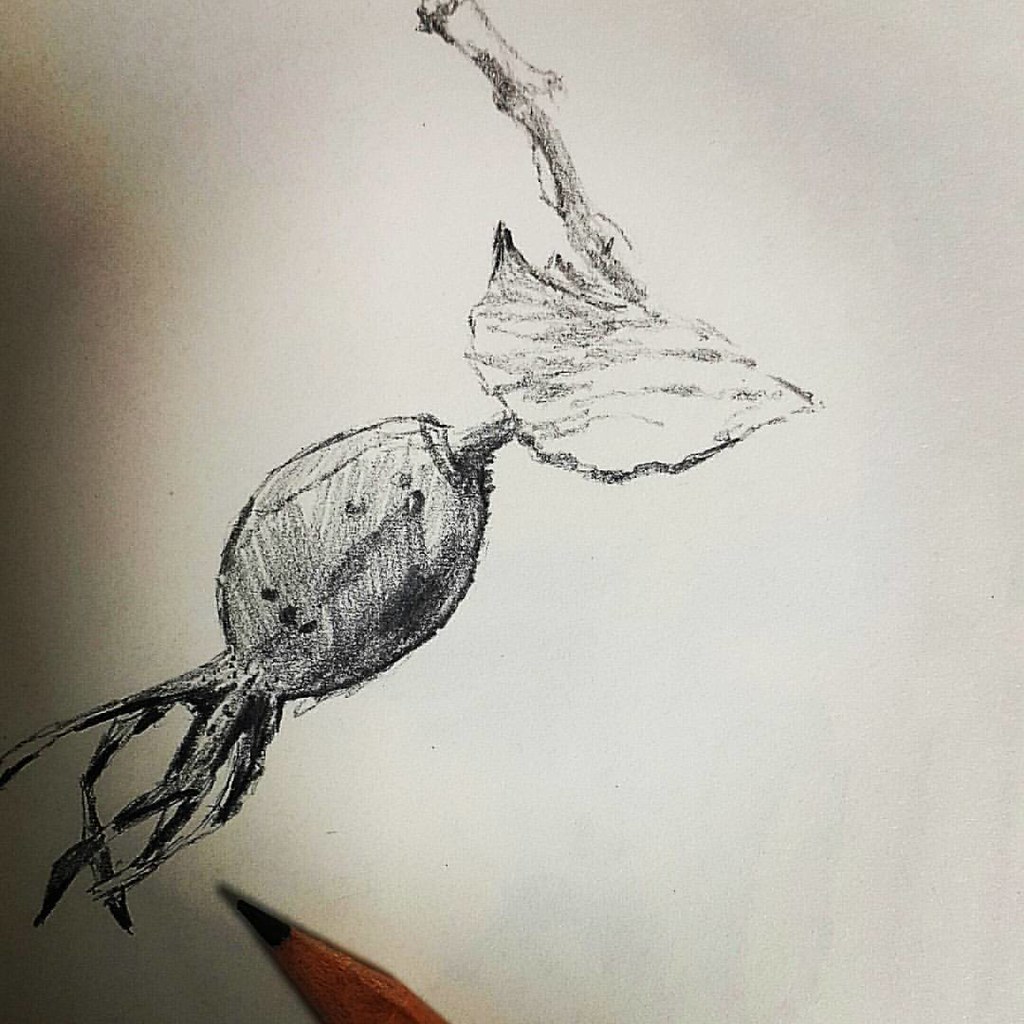A highly detailed, close-up view of a pencil drawing on white paper captures the viewer's attention. Positioned in the bottom left corner, one can spot the tip of the pencil likely used by the artist. The left side of the image is marked by a prominent shadow, adding depth and contrast to the composition. Central to the frame, the drawing itself emerges, though its subject is somewhat ambiguous. From the top center, a branch or twig appears to extend downwards, connecting to a round, bulbous object that resembles a piece of fruit or possibly a radish. This object features distinctive, spiky protrusions, enhancing its organic and slightly mysterious appearance.